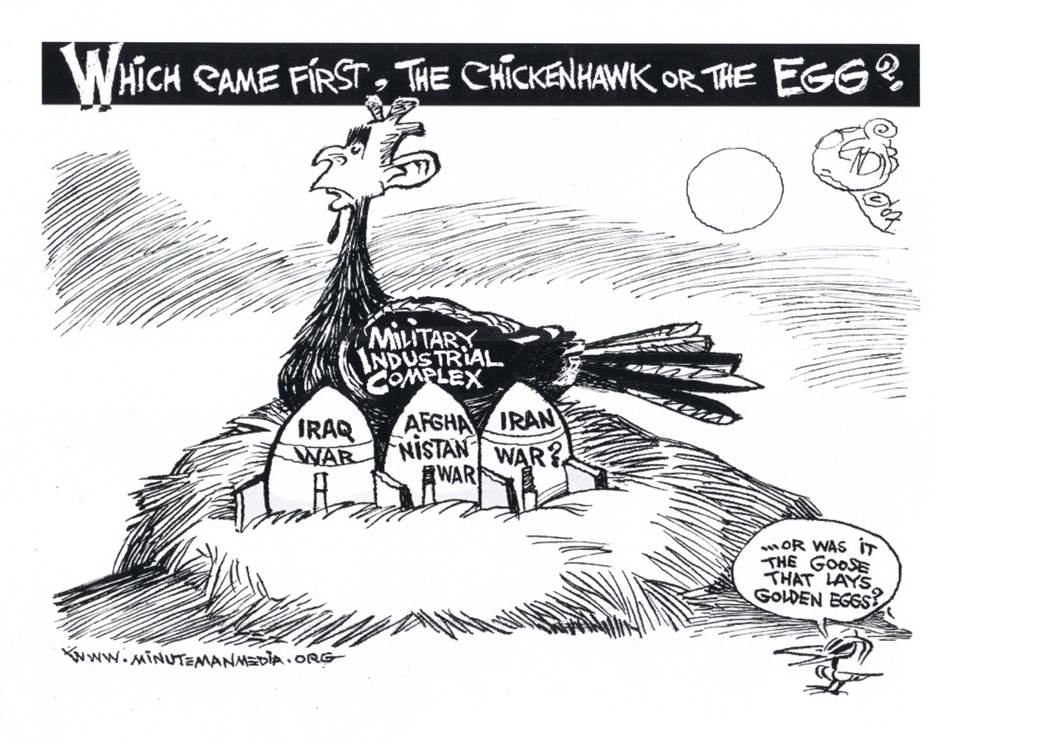The image is a comic-style cartoon with a black header and white text at the top that reads, "Which came first, the chicken, hawk, or the egg?" In the center of the image, there is a peculiar bird with the head of a person, representing the "military industrial complex," facing left. This bird is situated in a nest that holds three eggs, each labeled with a different war: Iraq war, Afghanistan war, and Iran war. In the bottom right corner of the image, there is a caption that asks, "Or was it the goose that lays the golden eggs?", next to a malformed bird resembling Tweety Bird with a long beak. This image is a detailed satirical commentary on the military industrial complex and the wars initiated, suggesting these conflicts are equated to the "golden eggs" for income generation.